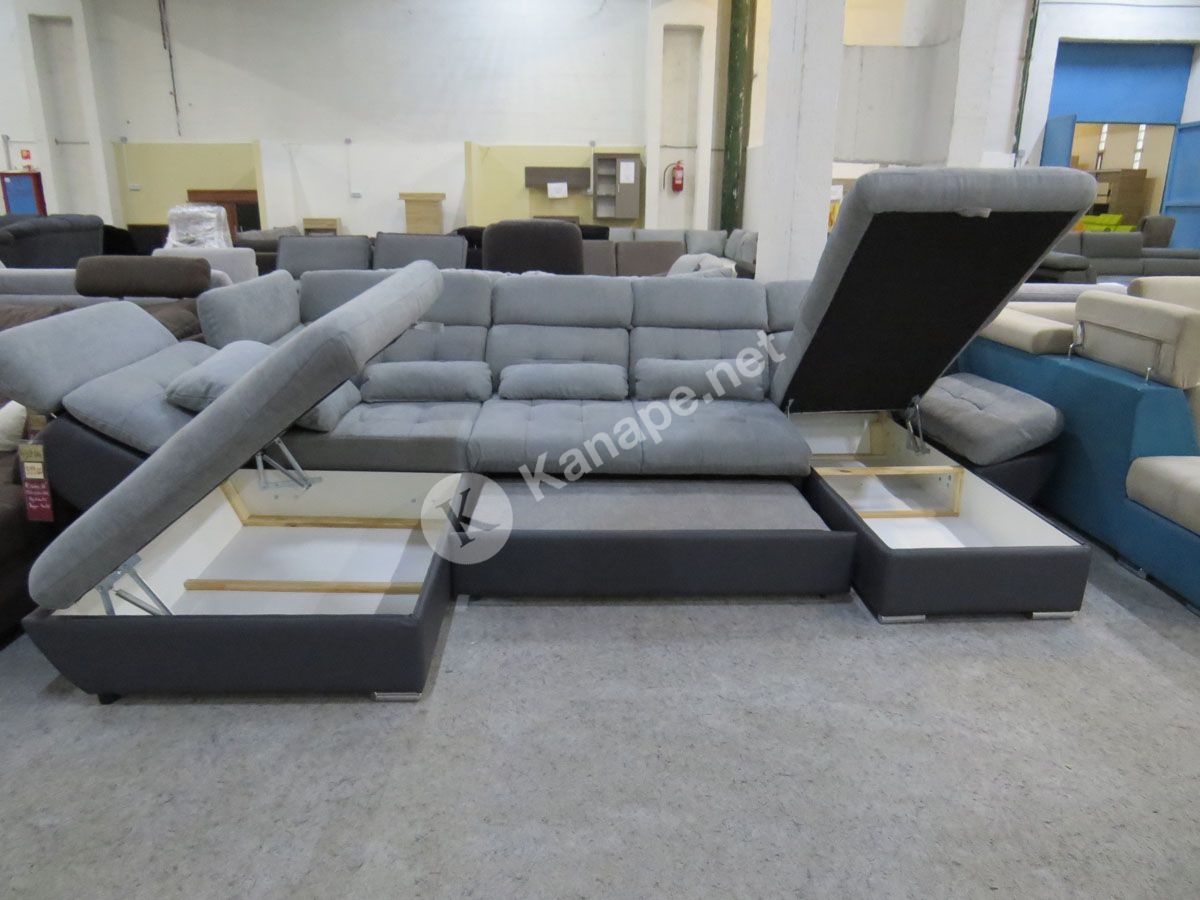The photograph captures the inside of a warehouse-style furniture store, specifically focusing on a highly functional grey sectional sofa prominently positioned on a grey carpet. The sectional, which is wider than it is tall, forms an L-shape with its longer side extending towards the right and then towards the viewer. The sectional is not just for seating—it offers extensive storage options. The right side of the L reveals a spacious storage compartment, accessible by lifting the seat, showcasing a white interior. Similarly, the left side also lifts to reveal an additional white storage space. Moreover, the center section of the sofa features a pull-out double bed, enhancing its versatility.

In the background, the store is filled with various other couches and chairs, including a mix of grey and a notable light brown couch. A red fire extinguisher is visible against a white wall, and a blue wall is in the top right-hand corner of the image. The photograph also includes a watermark in the center with the text "K-A-N-A-P-E.net" accompanying a logo. The overall ambiance is that of a well-stocked furniture showroom, ready for customers.